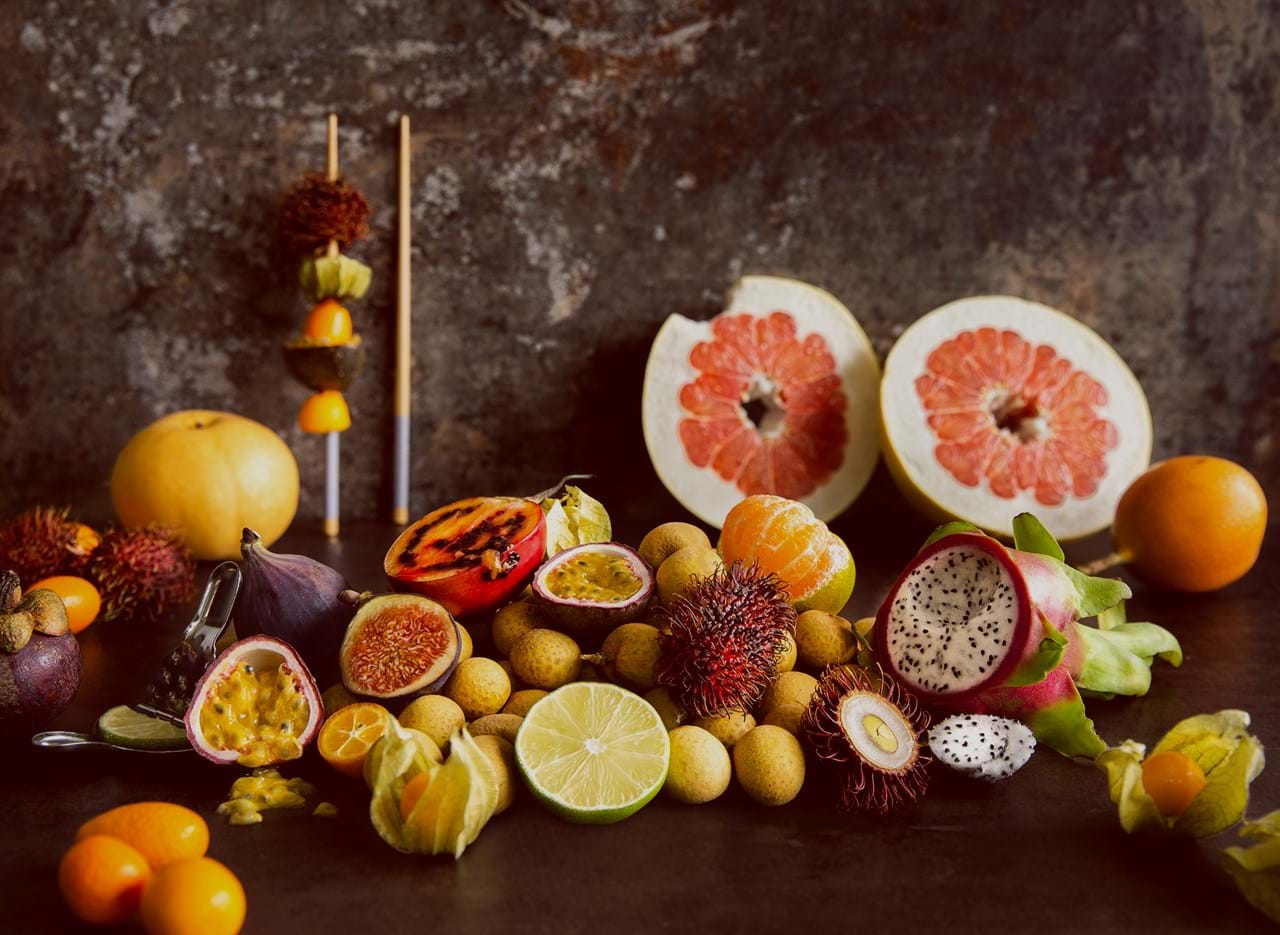This realistic photograph, horizontally oriented, depicts a vibrant and festive spread of various fruits meticulously arranged on a smooth, dark brown wooden table against a rough-textured, dark brownish-gray stone wall background. The table is adorned with a plethora of fruits in shades of yellow, green, orange, with a few red ones scattered throughout. Prominently featured are oranges, including a peeled one, a sliced lime, a pomegranate, star fruits, both whole and sliced revealing their small black seeds, and grapefruit halves showcasing their vibrant red interiors bordered by white. Among these are smaller fruits skewered and some fruits stuffed with a dressing. There are also kiwis, a tomato cut in half, grapes, and what appears to be some dried or drying fruits, possibly olives or small eggs. A small leaf plant is visible near a sliced orange on the far right, adding a touch of greenery to this bountiful, holiday-themed arrangement suitable for a festive centerpiece.